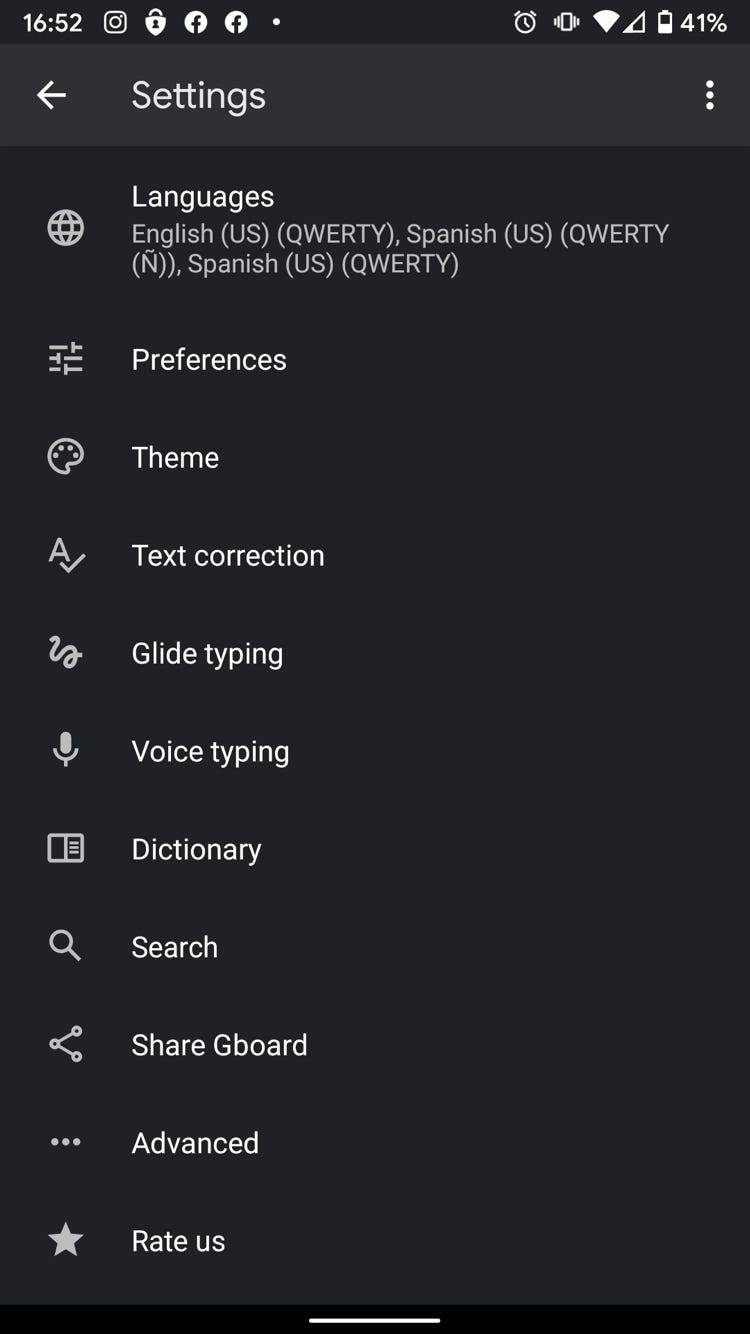This image is a detailed screenshot from a smartphone with a predominately black background. At the top of the image, the current time is displayed as 16:52. Surrounding the time are various icons including an Instagram icon, a lock icon, two Facebook icons side by side, a clock, Wi-Fi signal strength indicator, cellular signal strength indicator, and a battery icon indicating a 41% charge.

Directly beneath the status bar is a gray banner featuring a left-facing arrow next to the word "Settings" in bold lettering. Vertically aligned along the left-hand side of the screenshot are multiple menu options listed sequentially. These options include: Languages, with available selections of English (U.S.) and Spanish (U.S.), both using the QWERTY keyboard layout; Preferences; Theme; Text Correction; Glide Typing; Voice Typing; Dictionary; Search; Share; Gboard; Advanced; and finally, Rate Us.

The screenshot provides a clear and organized view of the phone's language and input settings menu, showcasing the extensive customization options available to the user.